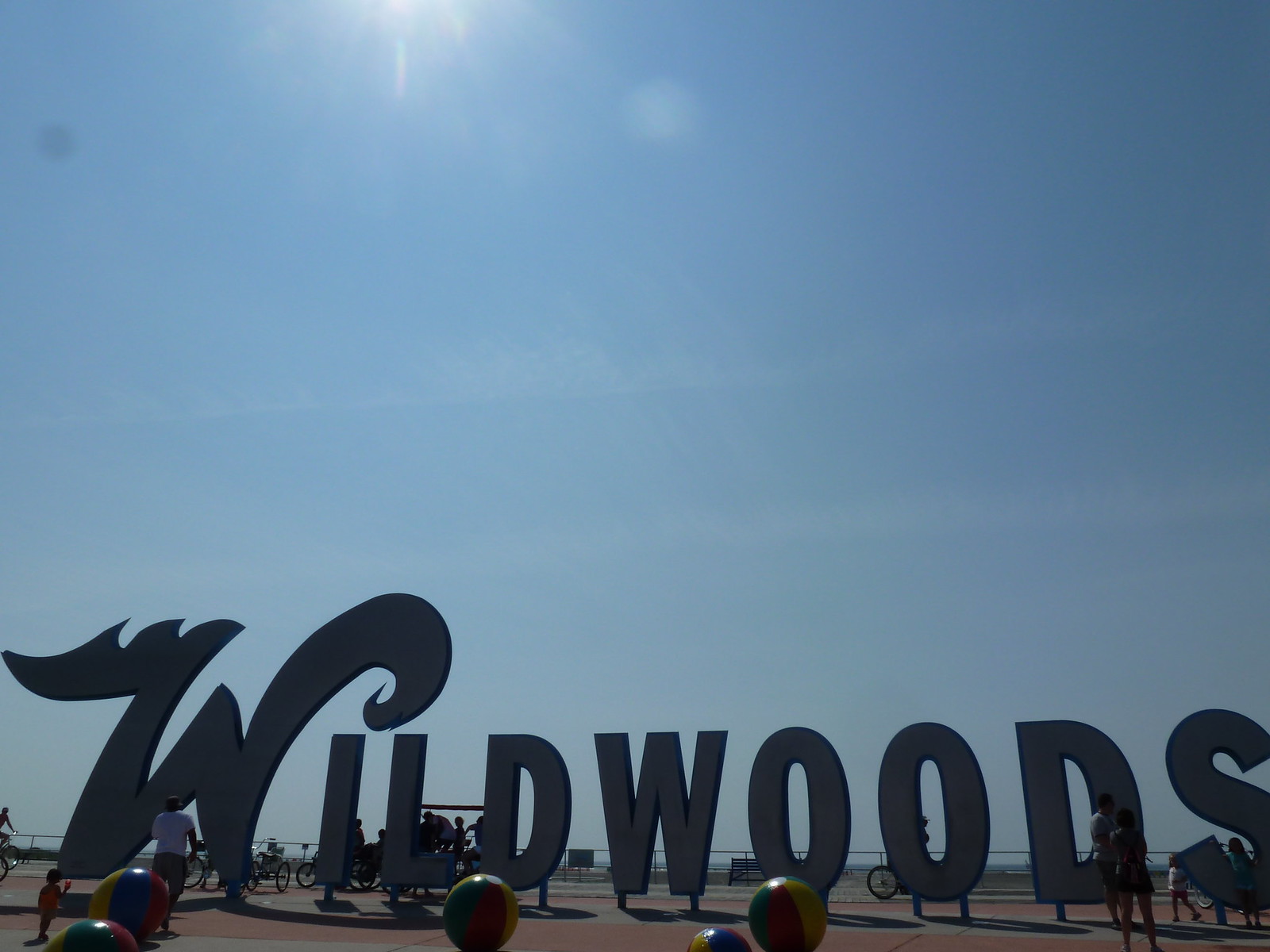This vibrant digital photograph captures an outdoor scene on a clear, sunny day with bright blue skies and just two small clouds. The focal point of the image is a large, prominent sign that spells out "Wildwoods" in individual letters. The first "W" is significantly larger and designed in a script font, contrasting with the more standard block letters of the remaining text. The scene appears to be set on a boardwalk or pier area, with several colorful beach balls (at least five) scattered in the foreground. 

In the background, numerous people are interacting with the area—some are standing, some are gathered around the sign, and one individual is taking a photo. There's a woman and a small child near the sign, with the child holding some food. Some kids are seen playing on the letters of the sign. Parked bicycles are visible behind the "W," and others are being ridden in the background. The image is awash with colors like blue, white, black, gray, green, yellow, and orange, capturing the lively and playful atmosphere of this park-like setting on a picturesque day.